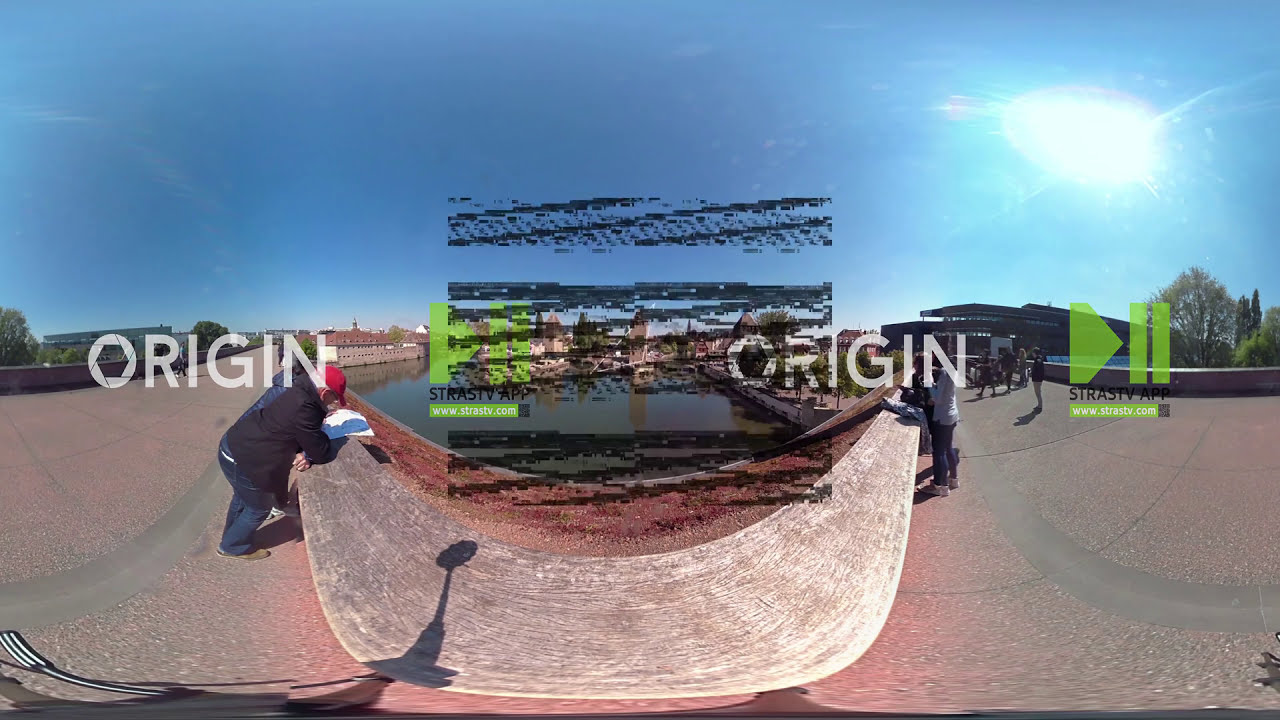The photograph appears to have been taken using a fisheye lens, causing a pronounced distortion that curves the image significantly. It shows an outdoor scene where people are resting on a horizontal structure, possibly a bench or railing, at a height that allows them to lean comfortably with their arms. These individuals seem to be looking out towards a body of water, although the water is not clearly visible due to heavy distortion and graphic overlays. 

The image has a central section with a graphic overlay, including text and symbols. On the left side and middle-right, the word "origin" is prominently displayed, with the 'O' resembling a camera aperture. Another green symbol resembling a triangle pointing right and two vertical bars, akin to Roman numeral II, is also present. Underneath these symbols, there's small black text that reads "STRASTV app", followed by more tiny white text on a green bar. 

In the background, over to the right, beneath a dark blue-purple sky with a glaring sun shining through clouds, there are housing structures or viewing stands. More people are visible, including a man in a red baseball cap, blue jacket, and jeans, seemingly examining some paperwork. The setting, which includes elements like a potential skateboard ramp and a dirt track, suggests a mixed-use, possibly recreational or competitive space.